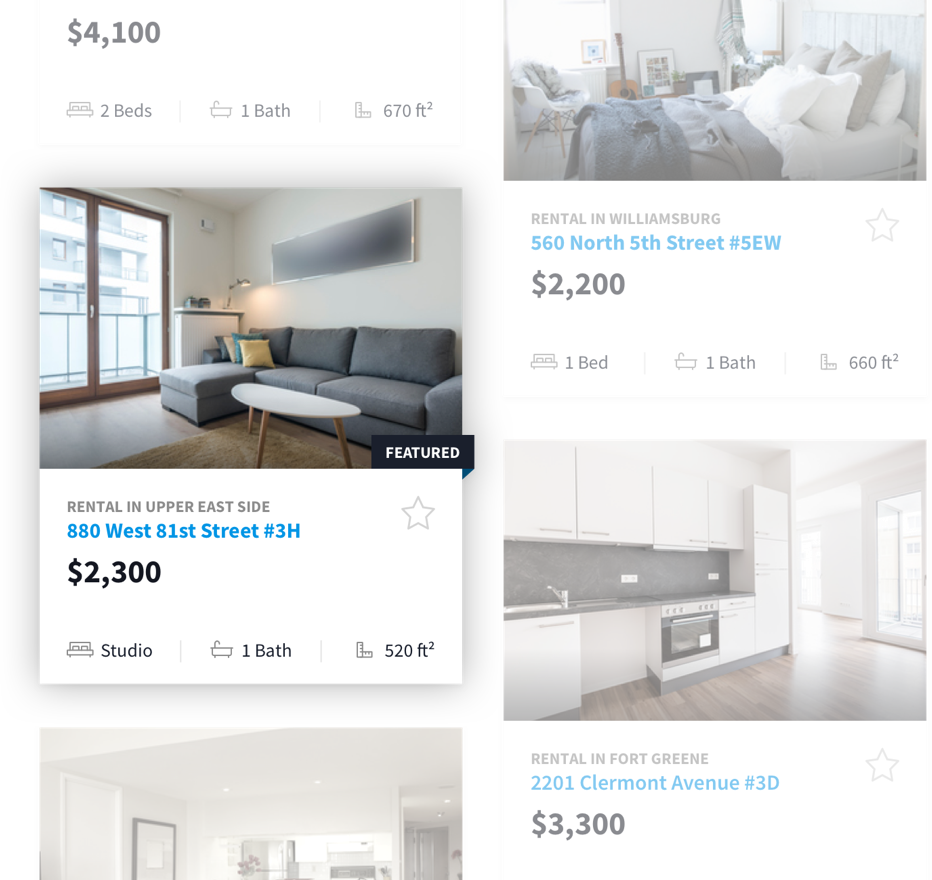The image appears to be a screenshot from a real estate website advertising various apartments available for rent. At the top left corner, although partially cut off, the price $4,100 is visible along with details indicating a unit with two bedrooms, one bathroom, and 670 square feet of space. To the right of this, there's a picture of a bedroom accompanied by information about a rental listing in Williamsburg at 560 North 5th Street, Unit 5EW, priced at $2,200 for a one-bedroom, one-bathroom apartment spanning 660 square feet.

On the left side, another listing shows a rental in the Upper East Side at 880 West 81st Street, Unit 3H. This section includes a picture of a living room and mentions a $2,300 studio apartment with one bathroom and 520 square feet. Lastly, the bottom right corner of the image displays an open-concept kitchen. This corresponds to a rental in Fort Greene at 2201 Claremont Avenue, Unit 3D, listed for $3,300.